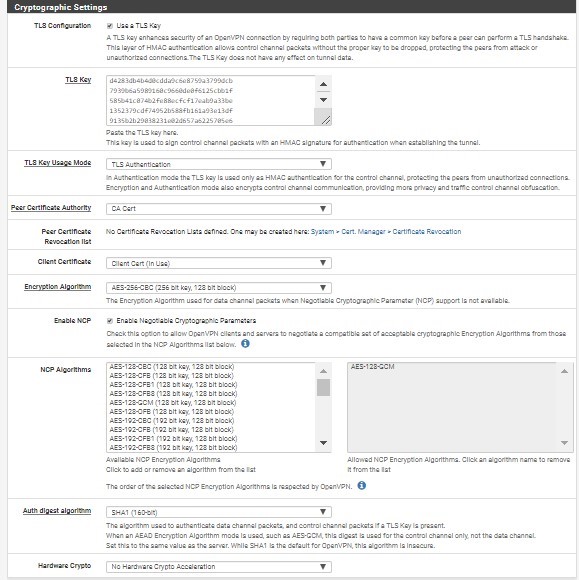Screenshot of a computer screen displaying cryptographic settings. At the top of the screen, the title "Cryptographic Settings" is prominently displayed, followed by a section labeled "Configuration". Underneath, there is the option "Use a TLS key as you go" accompanied by an explanatory paragraph. Further down, the setting titled "TLS Key" includes a rectangular input box with up and down arrows for adjustments. 

The next section, "TLS Key Usage Mode," features a drop-down menu, followed by "Peer Certificate Authority," which also has a drop-down menu. Below that is the "Peer Certificate Revocation List" option. Continuing downward, the "Client Certificate" section appears.

On the left side, various other cryptographic-related settings are listed, including "Encryption Algorithm" and "Enable NCP." The "NCP Algorithms" section features a drop-down menu for selection. Toward the bottom of the screen, there is the "Auth Digest Algorithm" setting, and at the very bottom, "Hardware Crypto."

Many of these areas contain input boxes, drop-down menus, and paragraphs of information. Several links, highlighted in blue, are present for further details or actions.